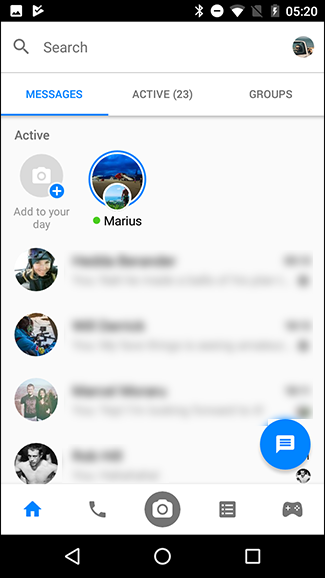This screenshot displays the interface of an Android phone, identifiable by the characteristic icons and the menu bar at the bottom of the screen. The topmost part of the interface features an empty search bar, and adjacent to it on the right, there is a profile picture, though its details are indistinguishable due to its small size.

Beneath the search bar are three tabs: "Messages," "Active," and "Groups." The user is currently on the "Messages" tab, highlighted in blue, while "Active" and "Groups" remain in dark gray. Just below these tabs, there is a section labeled as "Stories." The first option here is "Add to your story," represented by a gray icon featuring a camera image. Next to this, there is a story posted by someone named Marius.

Further down, various messages are displayed, albeit blurred out, with each message accompanied by a small icon. 

At the very bottom of the screen is the main navigation menu, featuring five icons from left to right: a house symbolizing the homepage, a phone icon presumably for calls, a camera icon for taking pictures, a bulletin list whose function is unclear, and a gaming console controller likely related to gaming features.

The time displayed in the top-right corner reads 5:20, without an indication of whether it is AM or PM.